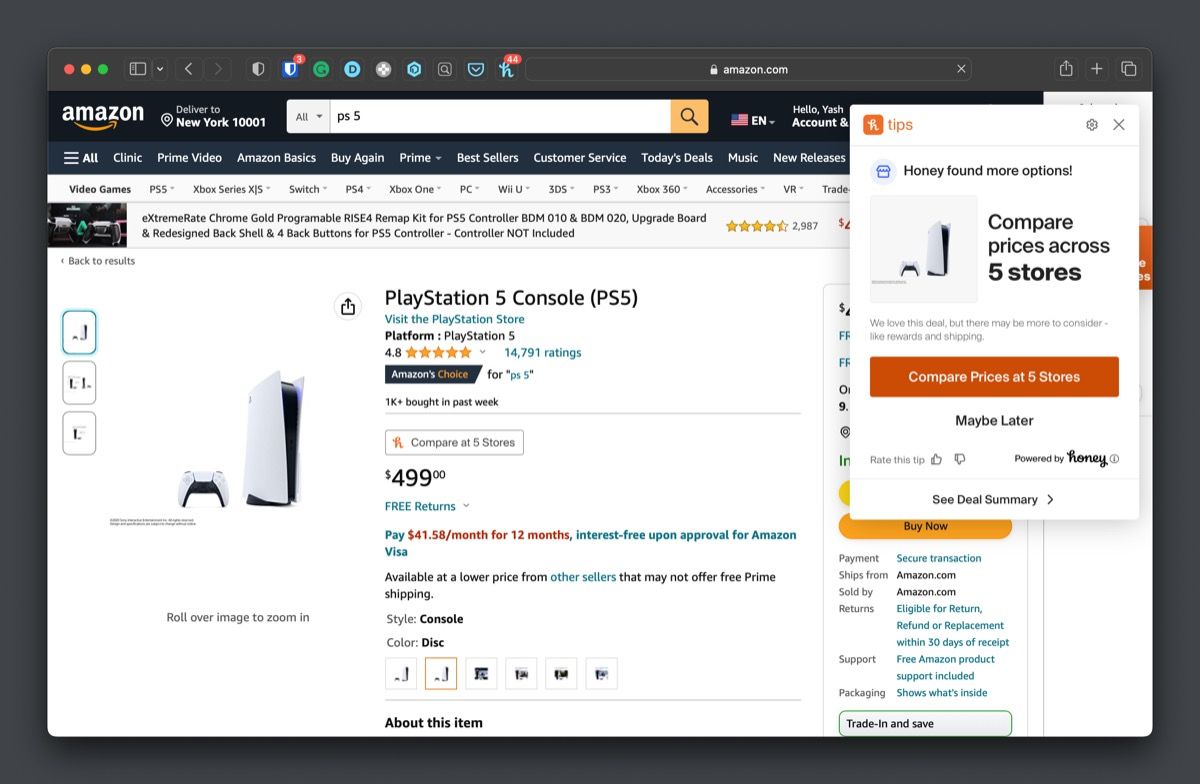In this image, a user is browsing Amazon on a Mac computer, as indicated by the distinctive red, yellow, and green window control buttons in the top left corner. The Amazon window has been resized to fit part of the desktop instead of occupying the entire screen. The user is viewing a product page for the "PlayStation 5 Console (PS5)" on Amazon. Below the product title, it prompts to "Visit the PlayStation Store" and specifies the platform as "PlayStation 5." The product holds a rating of 4.8 stars based on 14,791 reviews and is marked as "Amazon's Choice" for PS5, with a note that over 1,000 units were purchased in the past week. The listed price is a flat $499.00.

The product display adheres to the typical Amazon layout, featuring three selectable images on the left side of the screen. The currently displayed image shows the white PlayStation 5 console accompanied by a white controller positioned to its left. In the Amazon search bar above, the term "PS 5" can be seen, with an unusual space between "PS" and "5".

Additionally, there's a Honey extension pop-up on the right side of the screen, providing tips and alternative options. It mentions that Honey has found more options, offering to compare prices across five stores, with buttons labeled "Maybe later" and "See deal summary" at the bottom of the pop-up.